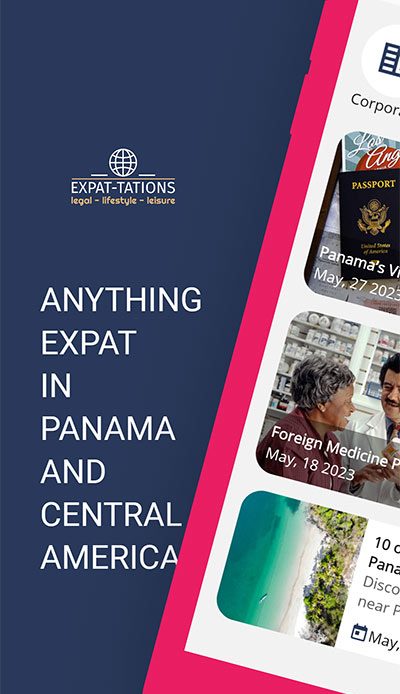This image is a promotional poster for "Expat-Tations" focusing on expatriates in Panama and Central America. At the top, a prominent globe symbolizes global connectivity, with the tagline "Anything Expat in Panama and Central America" beneath it. Just below, a smaller subtitle reads "Legal - Lifestyle - Leisure," emphasizing the diverse services and information available.

Diagonally across the poster are partially visible advertisements, beginning with a mention of "corporate services" alongside the date May 27th, 2023, accompanied by an image of a passport. The next segment features an older woman engaged in conversation with a pharmacist, labeled "Foreign Medicine" and dated May 18th, 2023.

The final section of the poster showcases an inviting beach scene with pristine white sand, bluish-teal water, and lush greenery. A beachside walkway invites exploration, with fragmented text reading "10, Panama, discover, near," and a partially visible date in May.

Overall, the poster effectively conveys the multi-faceted aspects of expatriate life, from legal and corporate services to healthcare and leisure activities, within the vibrant environments of Panama and Central America.